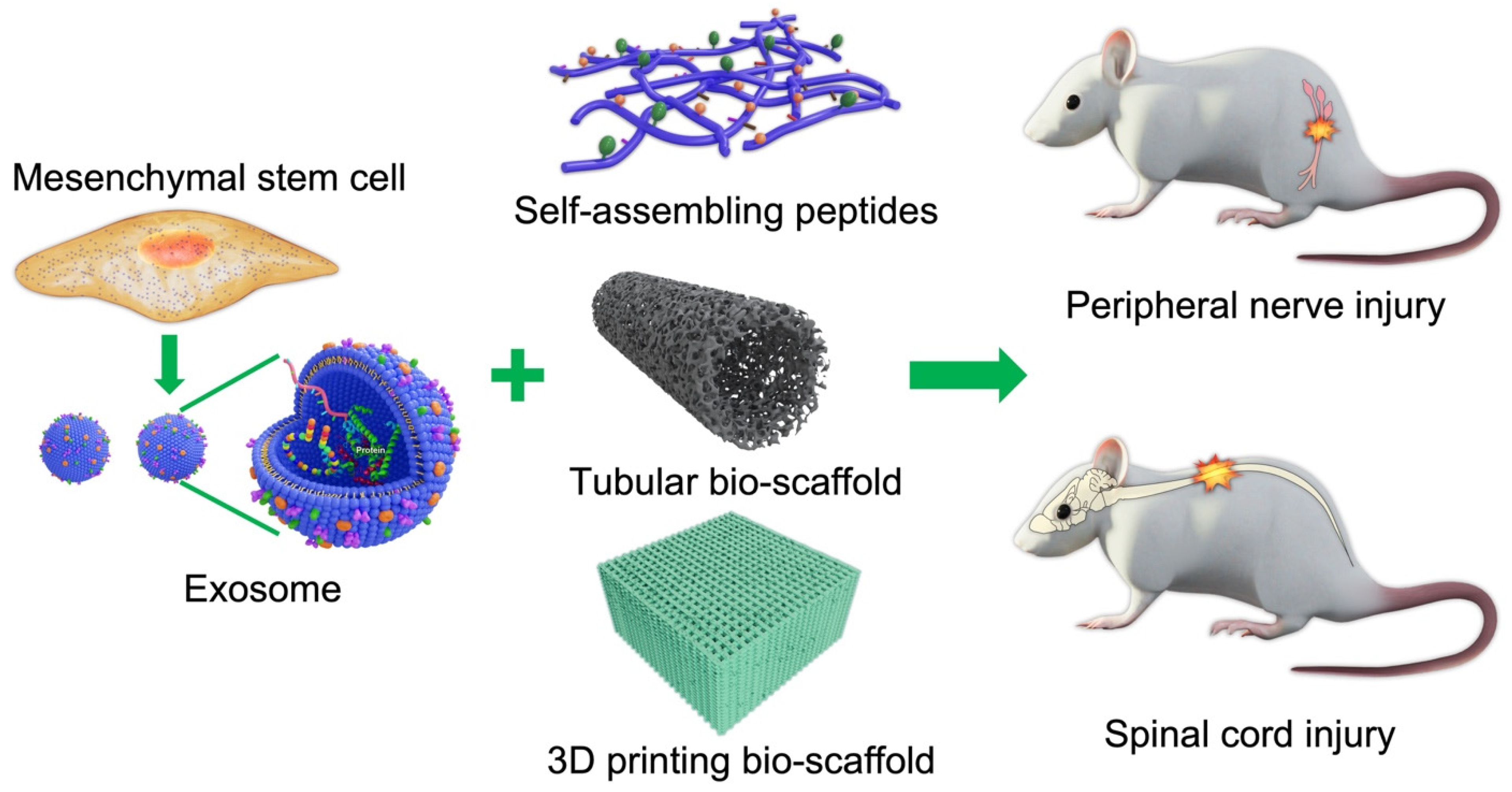The image shows a detailed flowchart from a textbook, illustrating the biological components and mechanisms involved in peripheral nerve injuries and spinal cord injuries using a white rodent model. On the right-hand side, there are two representations of mice: the top one highlights a peripheral nerve injury near the lower back, while the bottom one indicates a spinal cord injury closer to the upper spine. Arrows indicate the flow of biological processes and elements involved in the repair mechanisms.

On the left side of the flowchart, at the top, there is an image of a mesenchymal stem cell depicted as a yellow, oblong shape with black dots and a red circle in its center. Below this, an arrow points to two blue circles labeled as exosomes, one of which is cut open to show its internal structure.

Following the exosomes, the chart features several key components arranged vertically, connected by arrows. First, self-assembling peptides represented as red or purple tubes, followed by a tubular bioscaffold shown as a gray cell matter, and finally a 3D printing bioscaffold depicted as a square. The diagram includes plus signs to indicate the combined use of these components in treating the injuries.

This comprehensive illustration serves as a visual guide to understanding various aspects of both peripheral nerve injuries and spinal cord injuries, covering the involvement of stem cells, exosomes, and advanced bioscaffold technologies.